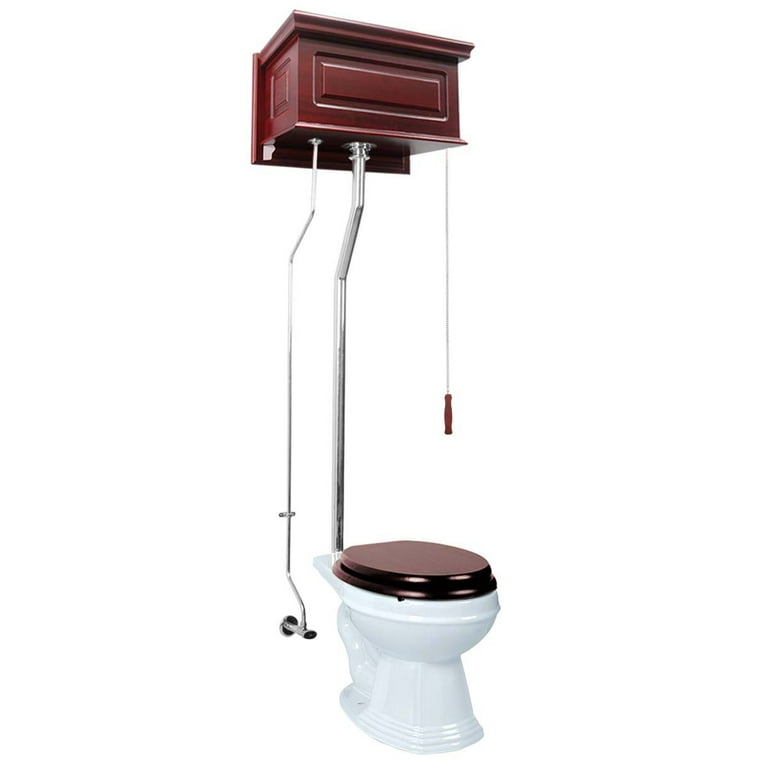This detailed, full-color photograph showcases an old-style toilet set against a stark white background, creating a frame-free vertical rectangle. The toilet bowl, likely porcelain, is white, complemented by a polished, dark brown wooden lid and seat. Above the toilet, a metallic pipe extends vertically from the toilet to a matching dark brown wooden cistern mounted on the wall. This cistern features a white pull chain with a dark brown handle, indicating the flushing mechanism. From the cistern, a thinner metallic pipe descends directly into the wall, presumably for water drainage. Additionally, there's a spigot near the toilet base for water flow control, attached to another pipe leading upwards to the cistern, indicating a complete flushing system.